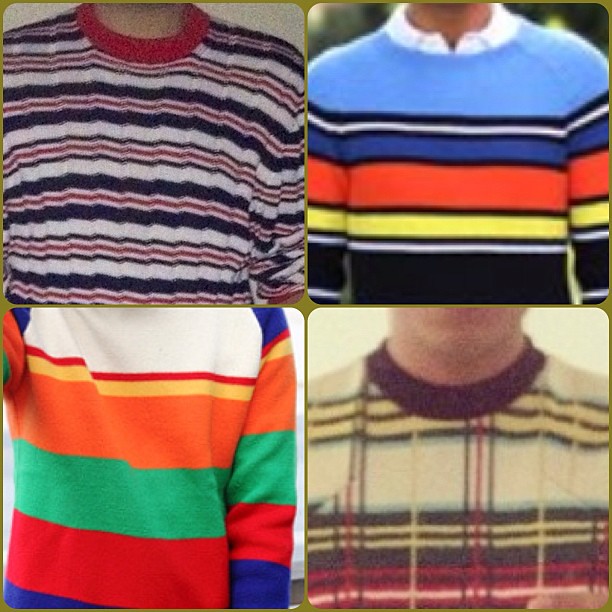The image is a vertically rectangular collage featuring four individual square photographs, each bordered in a greenish-gold color with rounded corners. All photos depict models wearing long-sleeved, striped sweaters shown from the neck down. The upper left photograph is quite grainy, showing a sweater with a red collar and horizontal stripes of navy, gray, and white with a thin red stripe in the middle. The upper right photo shows a clearer view with a light blue band across the shoulders and chest, followed by thin black, white, dark blue, orange, black, yellow, black, and white stripes, worn over a white button-down collar shirt. The background features an out-of-focus, outdoor green scene. The bottom left image only shows the torso and left arm of a model wearing a rugby-style sweater with broad stripes of white, red, yellow, orange, green, and blue. Finally, the bottom right photo is the fuzziest, revealing a sweater with a maroon collar and horizontal plaid patterns in cream, red, pink, maroon, yellow, and green. Only the lower face of the model is visible with part of their chin and neck showing.